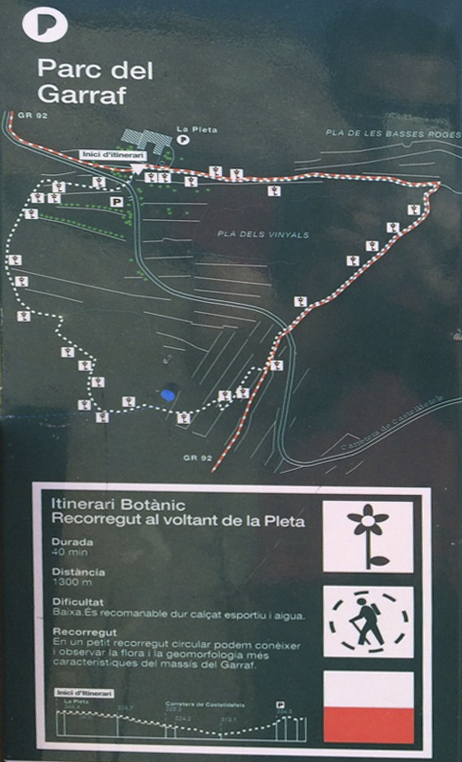The image is a portrait-oriented, color graphic map of a hiking trail in a foreign language. In the upper left corner, there is a white circle with a dark green stylized letter "P" inside. Beneath this, in white text, it says "Parc del Garraf." The top half of the image features a line art map of the trail, which includes various markers at points of interest denoted by white squares. The primary path of the trail is highlighted with alternating red and white horizontal lines, and there's a blue line suggesting a road that runs diagonally through the middle of the map. In the bottom half, a white-bordered panel displays text and symbols. To the right of this panel, there are three white squares containing trail symbols: the top square has a dark green flower, the center square shows a hiker in profile holding a staff and backpack within a broken line circle, and the bottom square is divided into a white half over an orange half. This detailed legend appears to provide information about the trail's features and duration, with labels such as "Dorada, 40 minutes distancia" indicating a 40-minute travel time and hints of difficulty. The black background has subtle variations in shade, possibly reflecting the paper's texture, adding to the overall style of graphic design and typography.